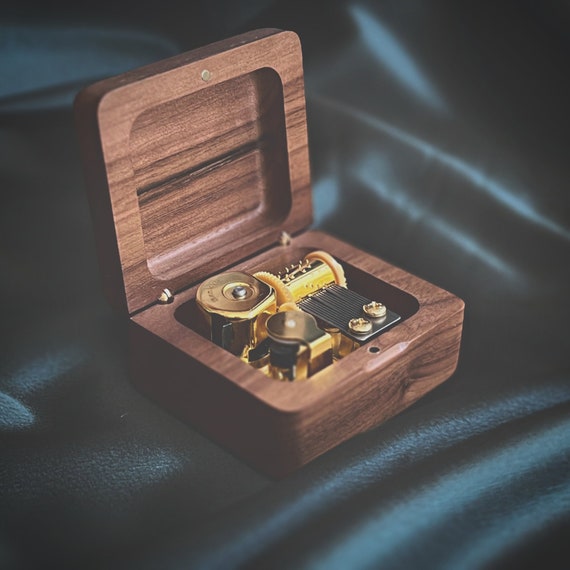This photograph depicts an intricately designed music box housed in a square-shaped, dark brown wooden case. The lid of the box is hinged open, revealing the complex inner mechanisms. The background features a greenish-aqua colored sheet, adding a contrasting element to the wooden box. Inside the box, various metallic components in copper, gold, and black are visible, with several gears, cylindrical pieces, and a mechanism designed to produce sound.

Central to the music box’s mechanism is a cylinder with evenly spaced components, likely responsible for striking different parts to generate musical notes. Some cylindrical parts, standing upright, seem integral to powering the device or ensuring its movement. Additionally, certain bolts and screws are also visible, contributing to the construction and functionality of the music box. The internal components rest within a shallow indentation on the base, with a possible shiny, black cloth lining at the bottom. This assembly of parts highlights the box’s purpose of creating music, emphasizing the craftsmanship and detail involved in its design.